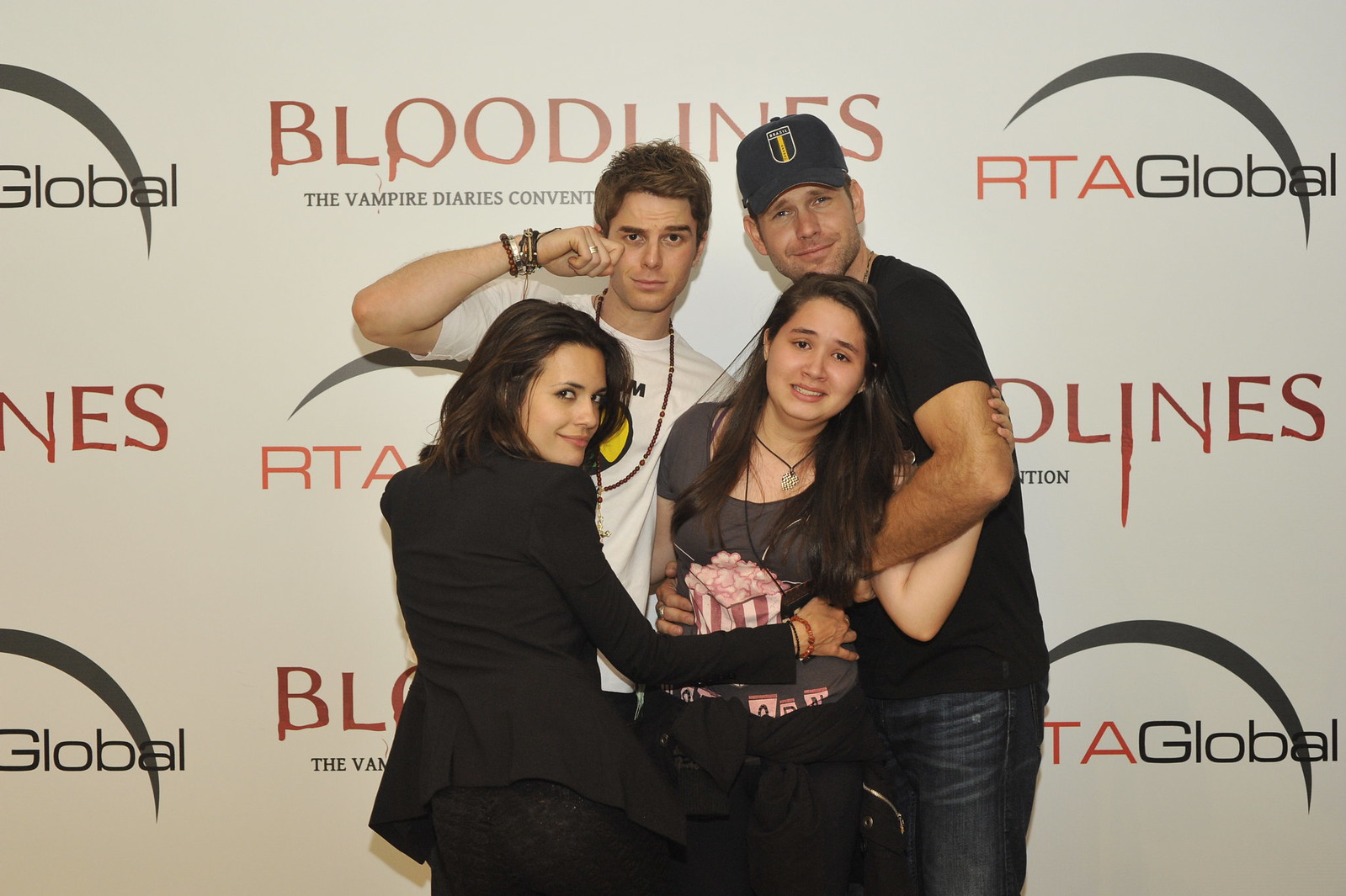In this image, four individuals are posed in front of a repeating backdrop that prominently features the logos for "Bloodlines, the Vampire Diaries Convention," and "RTA Global." The group consists of two women at the front and two men behind them, all seemingly connected through various embraces and gestures. 

On the left, a woman with dark brown hair styled in a suit jacket and black pants is smiling over her right shoulder at the camera. She is affectionately wrapping her right arm around the waist of another woman standing next to her. This second woman has long hair, is wearing a gray t-shirt with a cartoon drawing of a bucket of popcorn, and looks somewhat pained. She is being embraced from behind by a man dressed in a black t-shirt and jeans, sporting a black trucker cap with a yellow shield logo. His right arm is securely around her waist while his left hand is hooked over her arm. He, too, has a pained expression.

Next to them, another man, with short brown hair and dressed in a white t-shirt embellished with a logo and several necklaces, stands with his right arm slightly raised as if pretending to wipe away a tear. His expression is intentionally exaggerated, complemented by several bracelets adorning his wrist. The backdrop behind them is stark white, featuring repeating logos of "Bloodlines" and "RTA Global" patterned down the entire background.